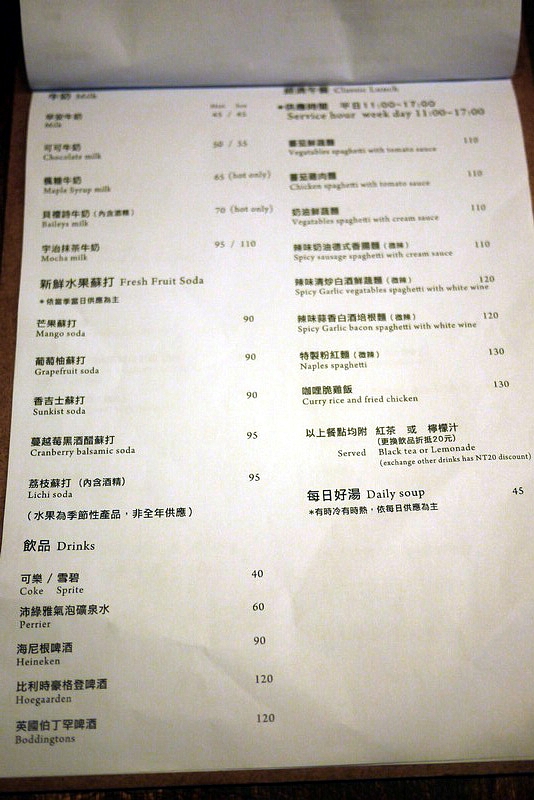The image captures an up-close view of a restaurant menu, although it is slightly blurry, making some parts difficult to read. The menu is formatted like a folded notepad rather than a book, with contents written in both Chinese and English. It lists various items along with their prices, without indicating the currency.

At the top of the left-hand column, the menu features a variety of drinks. Key highlights include:
- Plain Milk: $45
- Chocolate Milk: $50-$55
- Maple Syrup Milk (hot only): $65
- Bailey's Milk (hot only): $70
- Mocha Milk: $95-$110

The menu also lists fresh fruit sodas:
- Mango Soda: $90
- Grapefruit Soda: $90
- Sunkist Soda: $90
- Cranberry Balsamic Soda: $95
- Lychee Soda: $95

Further down, basic drinks are listed:
- Coke and Sprite: $40
- Perrier: $60
- Heineken: $90
- Hoegaarden: $120 (noted for possible misspelling)
- Boddingtons: $120

The right-hand column focuses on lunch options, particularly spaghetti dishes:
- Vegetable Spaghetti with Tomato Sauce: $110
- Chicken Spaghetti with Tomato Sauce: $110
- Vegetable Spaghetti with Cream Sauce: $110
- Spicy Sausage Spaghetti with Cream Sauce: $110
- Spicy Garlic Vegetable Spaghetti with White Wine: $120
- Spicy Garlic Bacon Spaghetti with White Wine: $120
- Maple Spaghetti: $130
- Curry Rice with Fried Chicken: $130

Noteworthy details include a note that lunch items are served with black tea or lemonade. Customers can exchange the drink for another option with a discount of NT$20. Additionally, the menu mentions a daily soup available for $45.

In summary, the menu from this Chinese restaurant attempts to accommodate English-speaking customers by providing bilingual descriptions and ensuring a variety of drink and meal options listed with corresponding prices.